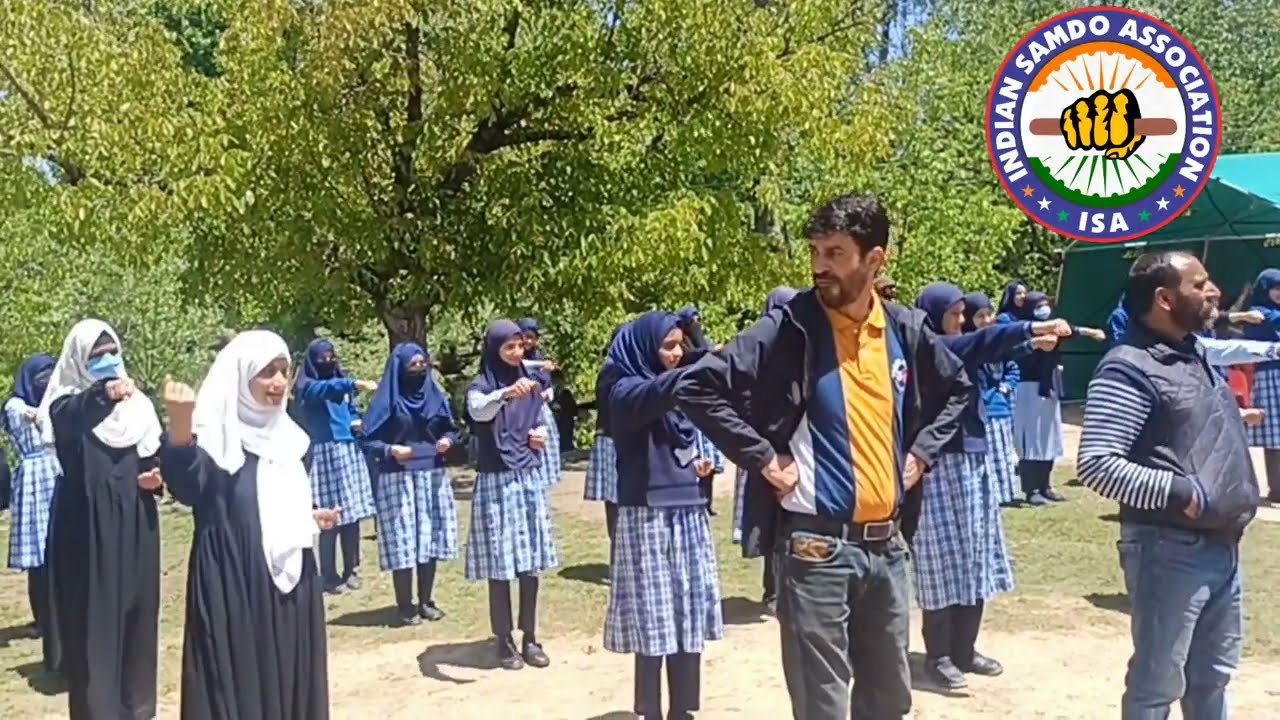In this photograph, a large group of individuals, mostly young females, are lined up in rows, appearing to participate in a coordinated activity organized by the Indian Sam Doe Association, as indicated by the logo featuring a hand wrapped around a pole and the text "ISA" in the top right corner. The setting is outdoors, in front of lush green trees. The young women predominantly wear blue plaid dresses, navy blue headscarves, and black pants. To the left, two women dressed as nuns in black tunics with white headscarves stand out. At the front of the lines are two men, one of whom is bearded and dressed in a blue hoodie, blue-striped shirt with gold accents, and jeans; he seems to be observing the activity. All individuals have their right arms extended straight forward with fists clenched, suggesting a synchronized exercise or ritual.